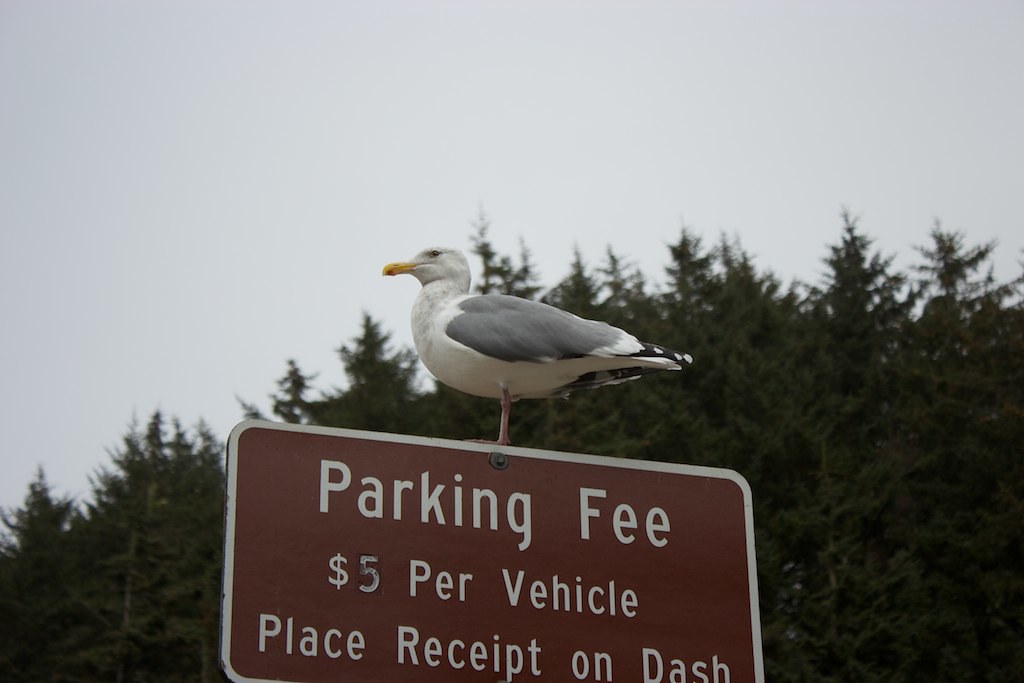The photograph captures a serene scene of a bird perched on top of a muted burgundy street sign with a white border and white lettering. The sign reads "Parking fee, $5 per vehicle. Place receipt on dash." The bird, which resembles a seagull, features a white body, gray and black wings, a yellow beak, and beige feet. The bird, looking placid and peaceful, faces to the left while standing prominently in the center on top of the sign. In the background, large dark green trees stretch out under a cloudy, gray sky.